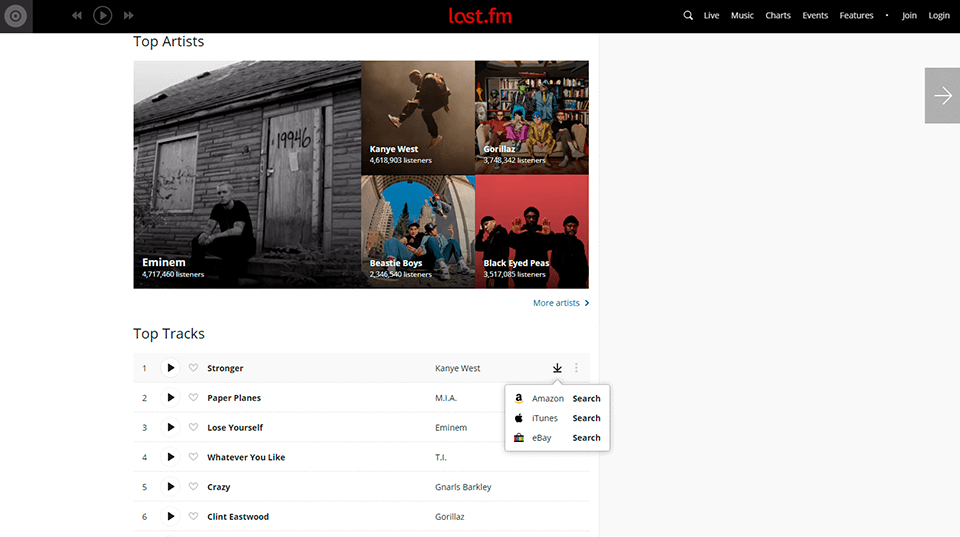**Screenshot Description of Last.fm Interface:**

This image is a detailed screenshot of a Last.fm user interface on a computer screen. 

1. **Top Navigation Bar:**
   - **Background**: Black fading to dark gray towards the left.
   - **Left Side**: Contains an icon with gray concentric circles and a central dark gray dot.
   - **Playback Controls**: Includes gray rewind, play (within a gray circle), and fast forward buttons.
   - **Center**: Displays the Last.fm logo in red text.
   - **Right Side**: Contains a white magnifying glass icon (search), followed by text links for "Live," "Music," "Charts," "Events," "Features," a dropdown arrow, and buttons for "Join" and "Login."

2. **Main Background**: Light gray and white.

3. **Top Artists Section**:
   - **Title**: "Top Artists" in black text.
   - **Artist Information and Thumbnails**:

     **Left Half**:
     - **Eminem**:
       - **Listeners**: 4,717,460
       - **Image**: Eminem sitting on a stoop in front of a block stone house with a boarded-up window on the left and a wooden door on the right with the number "19946" and a piece of paper attached to it.

     **Right Half**: Four artist thumbnails arranged in a square.
     - **Top Left**: 
       - **Kanye West**:
         - **Listeners**: 4,618,903
         - **Image**: Kanye West jumping in the air.
     - **Top Right**: 
       - **Gorillaz**:
         - **Listeners**: 3,748,342
         - **Image**: Four people on a tan sofa with a man standing behind, with bookshelves in the background.
     - **Bottom Left**: 
       - **Beastie Boys**:
         - **Listeners**: 2,546,540
         - **Image**: The group sitting with the Chancellor's Archway and a tall pine tree behind them.
     - **Bottom Right**: 
       - **Black Eyed Peas**:
         - **Listeners**: 3,517,085
         - **Image**: Three members against a red background.
     - **Text Link**: "More artists" in blue text.

4. **Top Tracks Section**:
   - **Title**: "Top Tracks" in black text.
   - **Track List** on a gray background: Contains track names with play button and heart icons next to them.
     1. "Stronger" by Kanye West (includes options to download via Amazon, iTunes, eBay, and a three-dot menu).
     2. "Paper Planes" by M.I.A.
     3. "Lose Yourself" by Eminem
     4. "Whatever You Like" by T.I.
     5. "Crazy" by Gnarls Barkley
     6. "Clint Eastwood" by Gorillaz

5. **Right Sidebar**:
    - **Large Light Gray Box** with a small dark gray box containing a white arrow pointing right.

The description captures both the visual composition of the Last.fm interface and the detailed textual content presented in the screenshot.